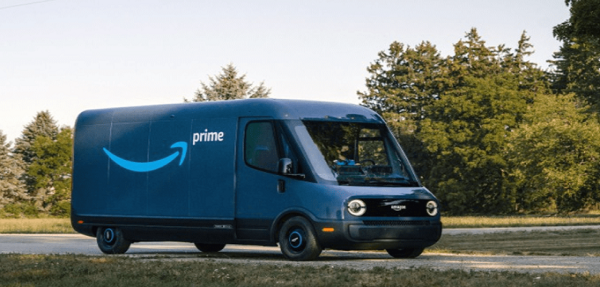The image captures an Amazon Prime delivery truck parked on a rural road. The dark blue vehicle, prominently displaying the Amazon logo and the word "Prime," is photographed at an angle, highlighting both the right side and the front. At the bottom of the image, a strip of grass suggests the truck is momentarily stationary. Seated behind the wheel is a solitary driver, who appears to be a man wearing a face covering. No other vehicles or individuals are visible in the frame, emphasizing the tranquility of the scene. The background is dominated by a dense array of trees, extending from the roadside up past the top of the photograph, further reinforcing the rural setting. The road is devoid of traffic, and there are no signs or text beyond the truck's branding, contributing to a sense of peaceful isolation.